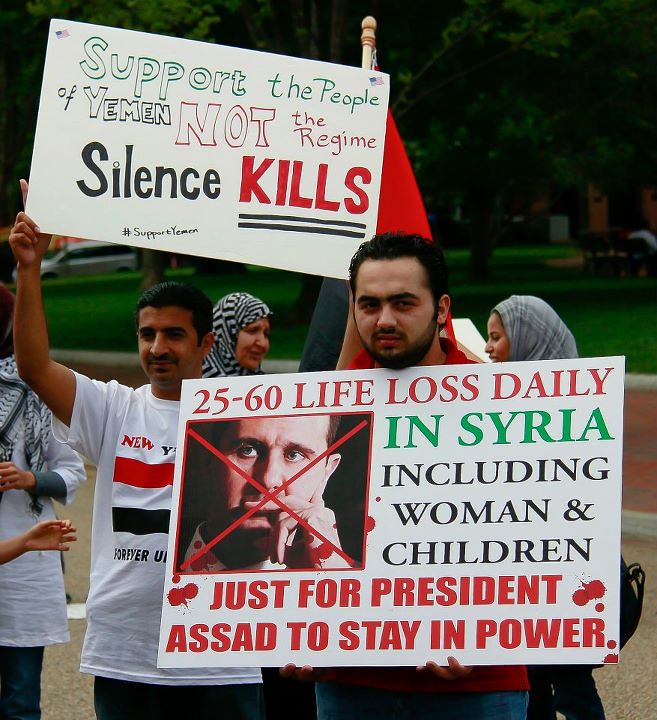This photograph captures a dynamic outdoor protest event against the regimes in Syria and Yemen. Central to the image is a bearded man, appearing in his late 20s to early 30s, holding a prominently displayed sign. The sign details the daily loss of 25 to 60 lives in Syria, including those of women and children, with a stern message directed at President Assad, whose photo features a large red X across it. Accompanying him is another man, dressed in a white shirt with red and black stripes, holding up a sign that reads in green letters, "Support the people of Yemen, not the regime. Silence kills." Additionally, two women in burqas, likely in their early 20s, stand behind them, seemingly engaged in conversation. The backdrop is a well-maintained green park with benches and trees, indicating the protest might be taking place on a campus or near a government building. Their assembly, highlighted by an overcast sky, showcases their solidarity in advocating for human rights and justice.